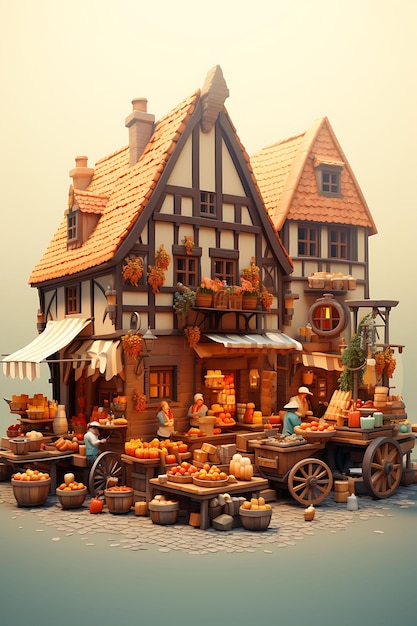The image showcases a detailed, computer-generated 3D scene featuring two medieval or early modern-style houses at the center, reminiscent of a German village. Both houses are adorned with gold cobblestone roofs, each roof having multiple chimneys—one red and one gray—and overlapping eaves. The buildings are framed with wood and have wood windows minus the glass panes. The house on the right has several distinct features: a dormer window, a small window ledge with baskets of orange flowers, and an awning above the door. The front facade sports one upper window, followed by two lower windows, and a small shelf outside. Inside, the store appears lit, showcasing indistinct items.

In front of the houses, a vibrant market scene unfolds, with tables loaded with an array of fruits and vegetables like pumpkins, apples, potatoes, and oranges. Wooden carts and baskets are packed with produce, adding to the bustling atmosphere. The cobblestone ground ties the scene together, contributing to the quaint, historical ambiance. People, presumably figurines, are depicted both behind the market tables, attending to the stand, and in front, browsing and shopping. The intricate detailing suggests this image could serve as a setting for a model train layout, likely O scale, emphasizing the meticulous craftsmanship in every element of the scene.